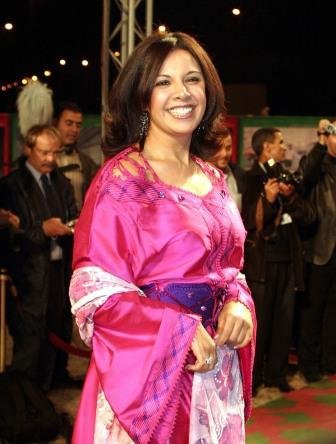In this indoor event image, a smiling brunette woman stands at the center, wearing a light pink formal dress accented with a cream-colored belt wrapped around her elbows and held in front of her. The dress features floral patterns, making her the focal point of the photograph. Surrounding her is a carpeted floor leading to a background filled with a group of photographers, some in dark suits and ties, while one is in a lighter suit. Though the photographers are largely focused on other subjects, one is distracted on his phone, and another is conversing with a colleague. Behind the woman, strands of light bulbs and a metallic column supporting the structure are visible, adding to the ambiance of the dimly lit room. The atmospheric lighting, combined with the array of colors—black, white, gray, yellow, red, pink, and purple—contributes to the sophisticated party setting captured in the middle of the night.